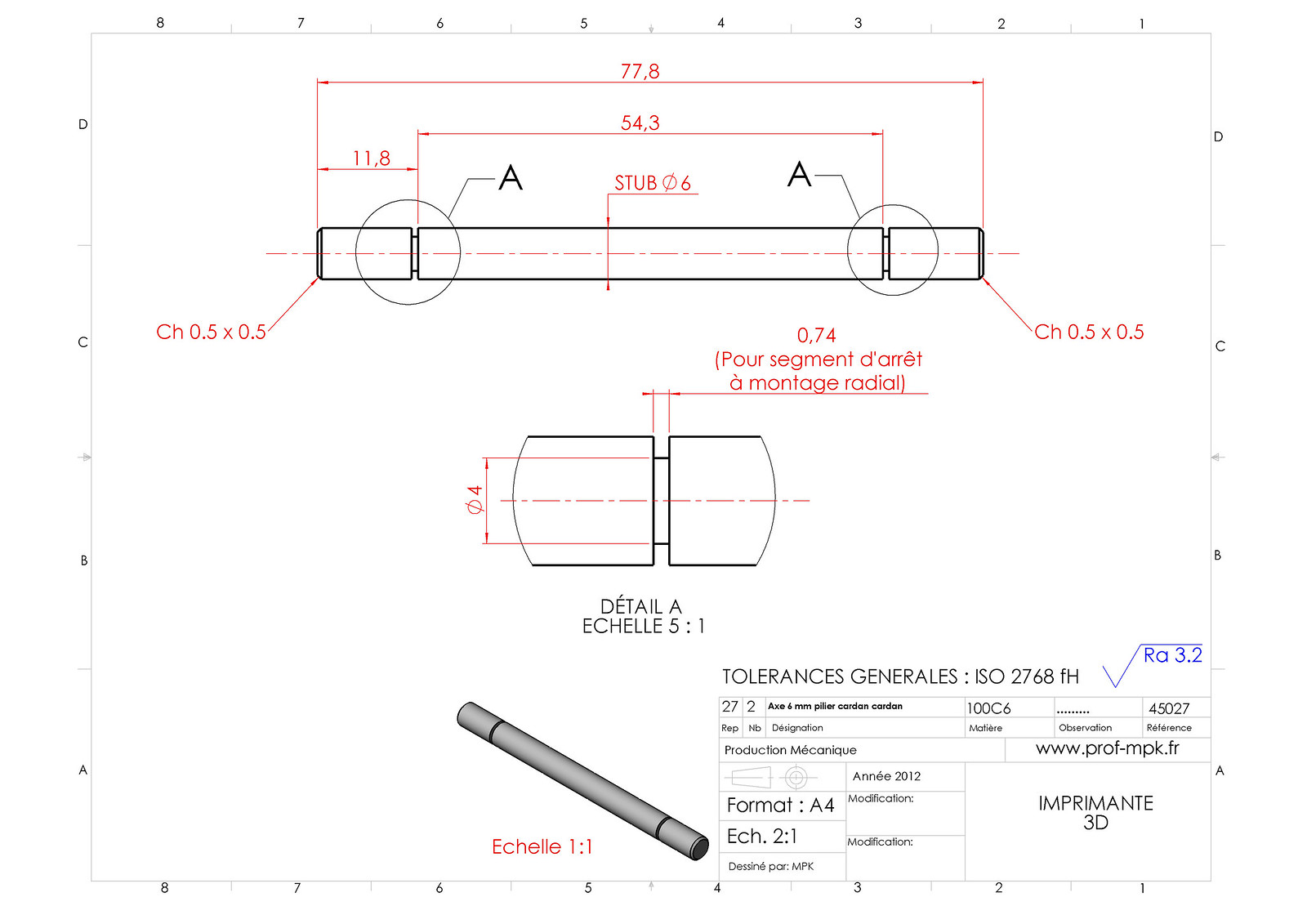The image is a detailed schematic, possibly of an electrical device or piping system, displayed on a rectangular white page. Along its borders, the top and bottom edges are consecutively labeled with the numbers 8 to 1 from left to right. Both the left and right edges are labeled with the letters D, C, B, A from top to bottom. The schematic itself, colored in red and black, features numerous labeled segments, the majority of which are annotated in French. Each segment is marked with its length. There is also a key or legend in the bottom right corner that likely provides additional information, such as part numbers or specific details about the schematic. A small box at the bottom includes a website: www.prof-mpk.fr.